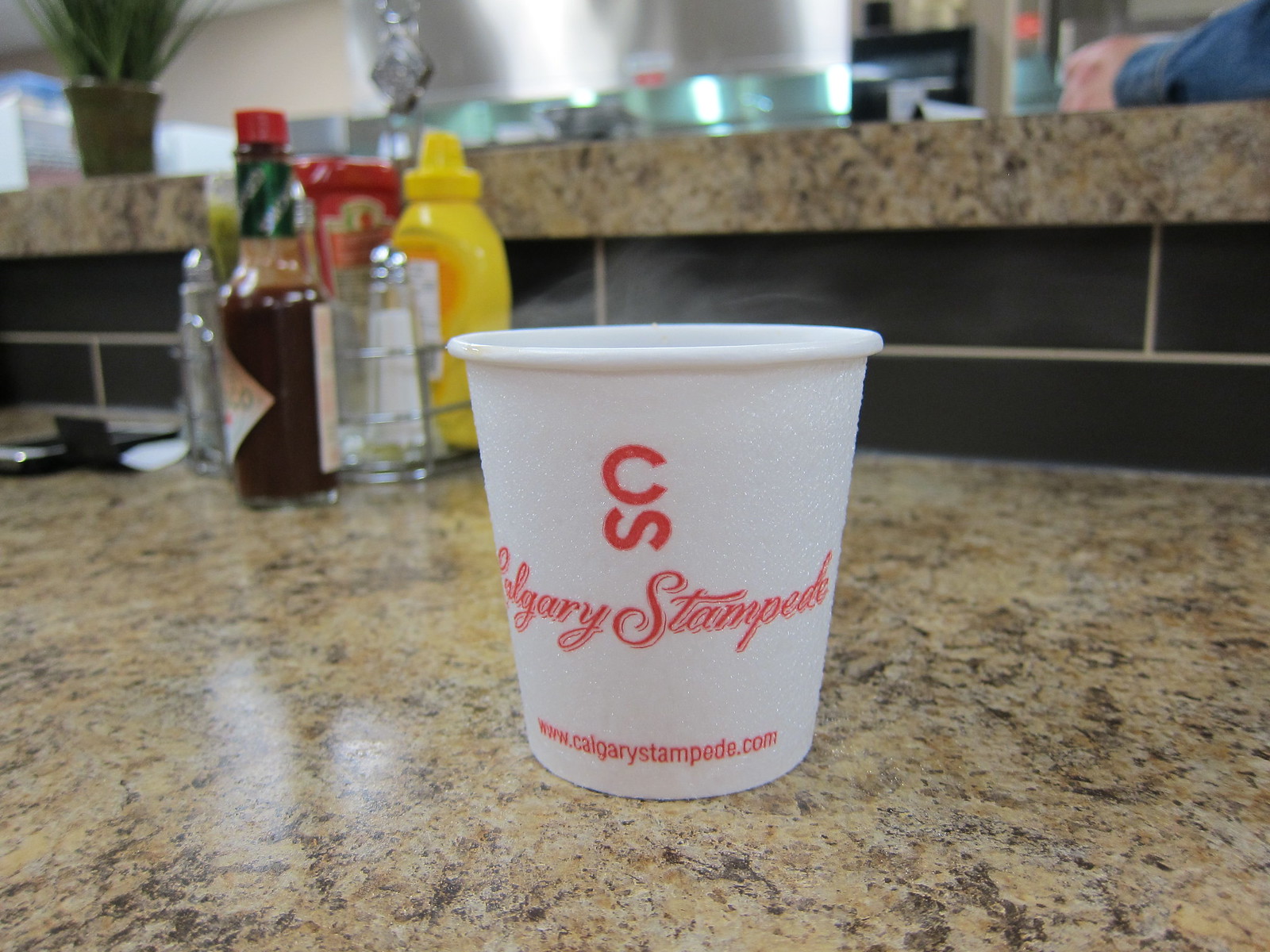This photograph captures a white styrofoam cup prominently displayed on a marbled countertop, blending shades of brown and dark brown. The cup bears the red letters "CS" followed by "Calgary Stampede" in matching red text, along with the website "www.calgarystampede.com." To the left and behind the cup, there is a collection of condiments, including mustard, Worcestershire sauce, salt, and pepper, with possible bottles of ketchup and Tabasco. The background reveals a higher level counter in black and white granite, which separates the foreground from a blurred scene beyond, featuring a counter and the indistinct arm of someone in a blue denim shirt or jacket.